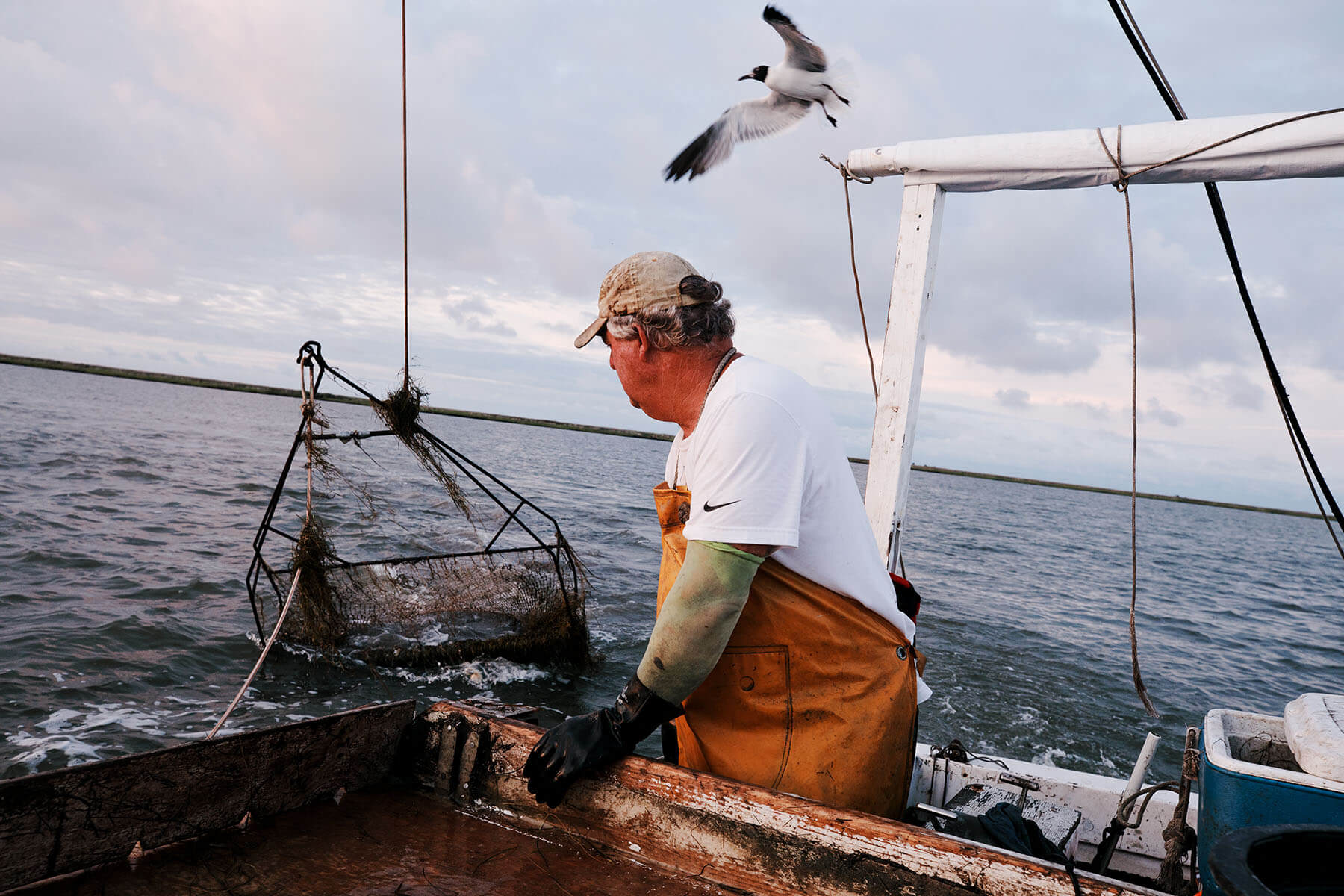In the image, a man engaged in crabbing is prominently featured on a rusted boat with a dark brown maroon floor. He is wearing a baseball cap and a protective orange raincoat over a white Nike shirt, complemented by long black gloves that reach mid-arm. The man, seen in a side view, is in the midst of pulling up a cage connected by an extended line. He also wears a brown apron. The boat's deck appears dirty, with a visible blue Igloo cooler nearby. Above, a black-and-white seagull hovers with outstretched wings. The backdrop features a vast, wave-accented blue body of water stretching to a distant, dark green landmass. The sky overhead is mostly gray with patches of white and blue, indicating a cloudy day.